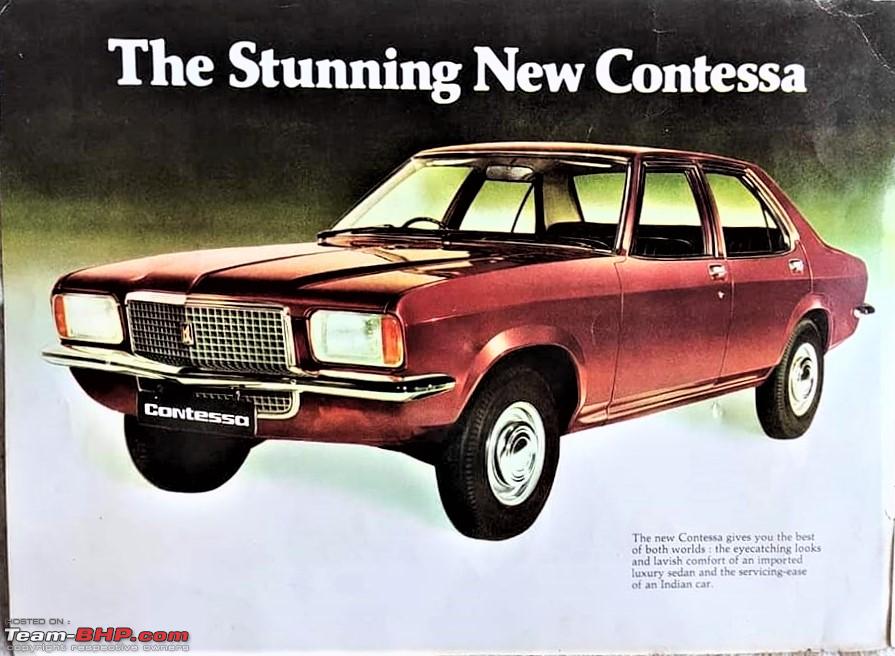This image is a wide advertisement that appears reminiscent of an old magazine or poster. It showcases the striking new Contessa, a classic four-door vehicle with a boxy design painted in an orangish-red color. The car is angled towards the left side of the image, highlighting its front grille, black tires, and silver wheels. The car features square or rectangular headlights with rounded corners and a silver grid-like grille with an emblem at the center. Below the grille is a black license plate displaying "Contessa" in white lettering.

The top portion of the ad is predominantly black, transitioning into a greenish-yellow color, finally blending into white at the bottom. In white text at the top, it reads "The stunning new Contessa." The bottom right corner includes a paragraph in black text, stating, "The new Contessa gives you the best of both worlds: the eye-catching looks and lavish comfort of an imported luxury sedan, and the servicing ease of an Indian car." Additionally, the ad mentions that it is hosted on Team BHP, with "Team" in white and "bhp.com" in red.